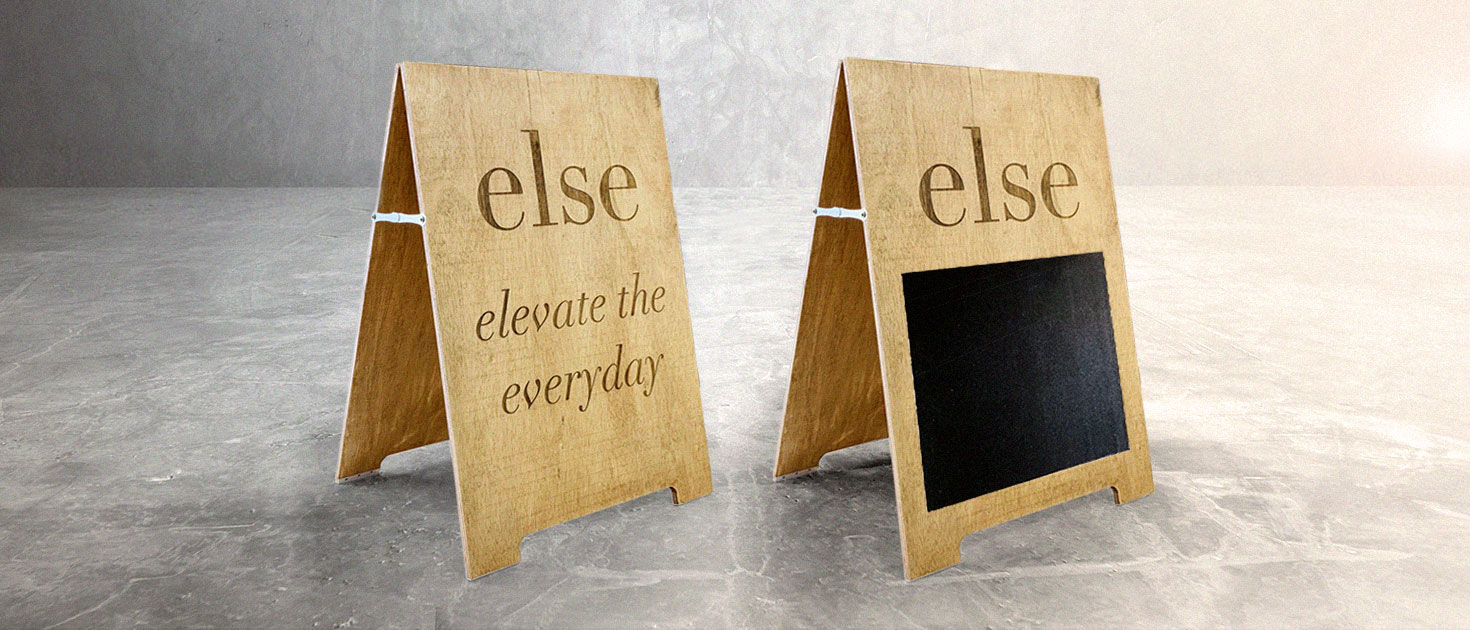This photograph, taken indoors, captures two triangular wooden signboards centrally positioned against a gray stone tile floor and a gray-painted wall. The signboards, which resemble easels typically used outside businesses to display messages, stand on light brown wooden legs with metal clips allowing them to fold for easy storage. The left signboard features text neatly etched in lowercase letters, reading "else" at the top and "elevate the everyday" beneath it. Meanwhile, the right signboard mirrors the design of its counterpart but includes a pitch-black rectangular area, reminiscent of a blank chalkboard, without any additional text. The lighting from the right casts a subtle peachy tone onto the gray backdrop, enhancing the simple yet sophisticated presentation of the wooden message stands.